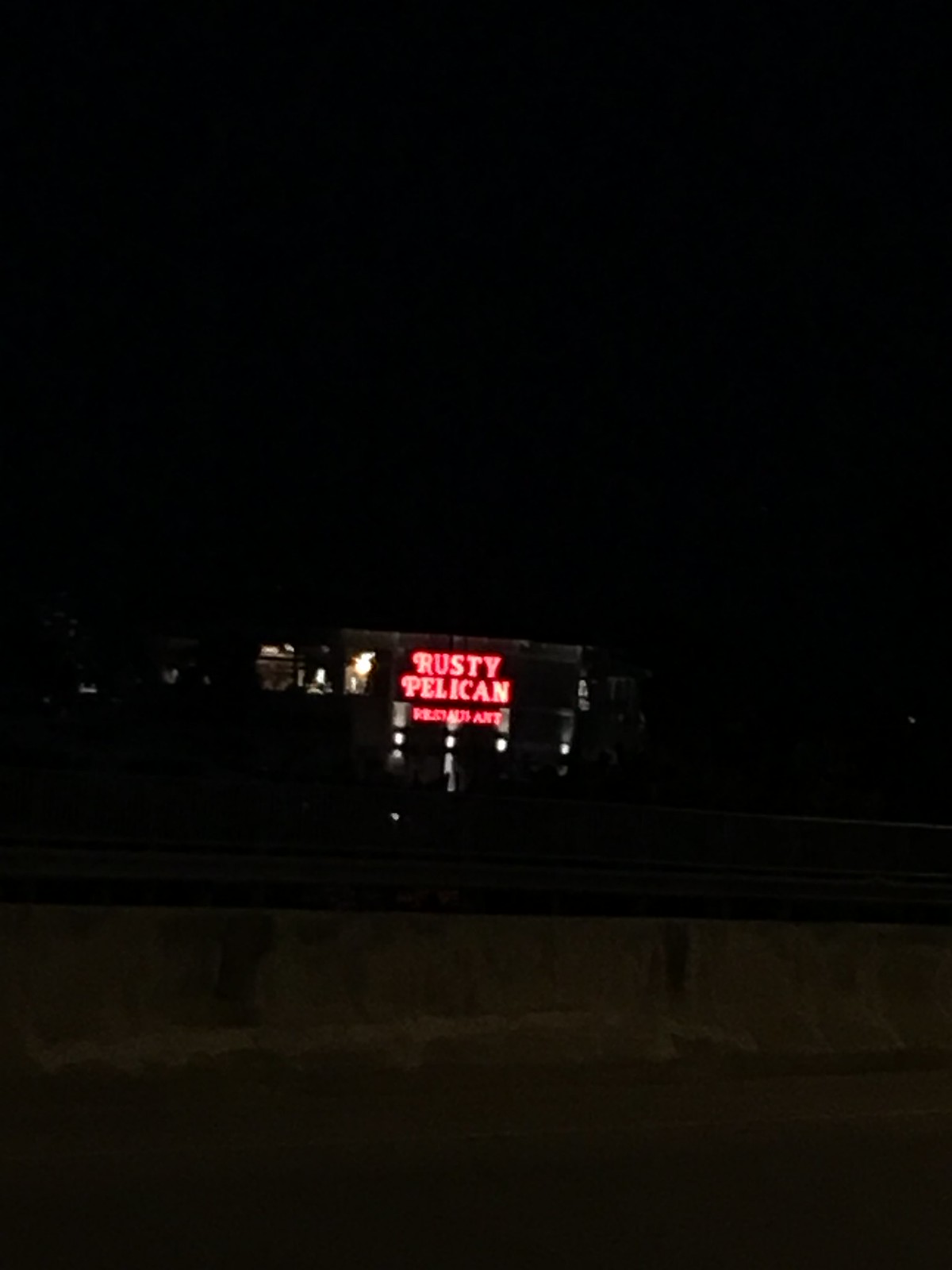The night-time photograph captures a moody, dark scene set outdoors. The sky is entirely black, and in the distance, there's a prominent billboard with a dark background. The billboard features the name "Rusty Pelican" in bold, bright red letters, with the word "Restaurant" displayed underneath in smaller red font. Various white lights illuminate the base of the billboard, enhancing its visibility and drawing attention. In the foreground, a low stone wall with a black top is visible, and what appears to be water crashes against it, adding a dynamic element to the otherwise still night. Despite the darkness, the photo conveys a sense of atmosphere and intrigue.